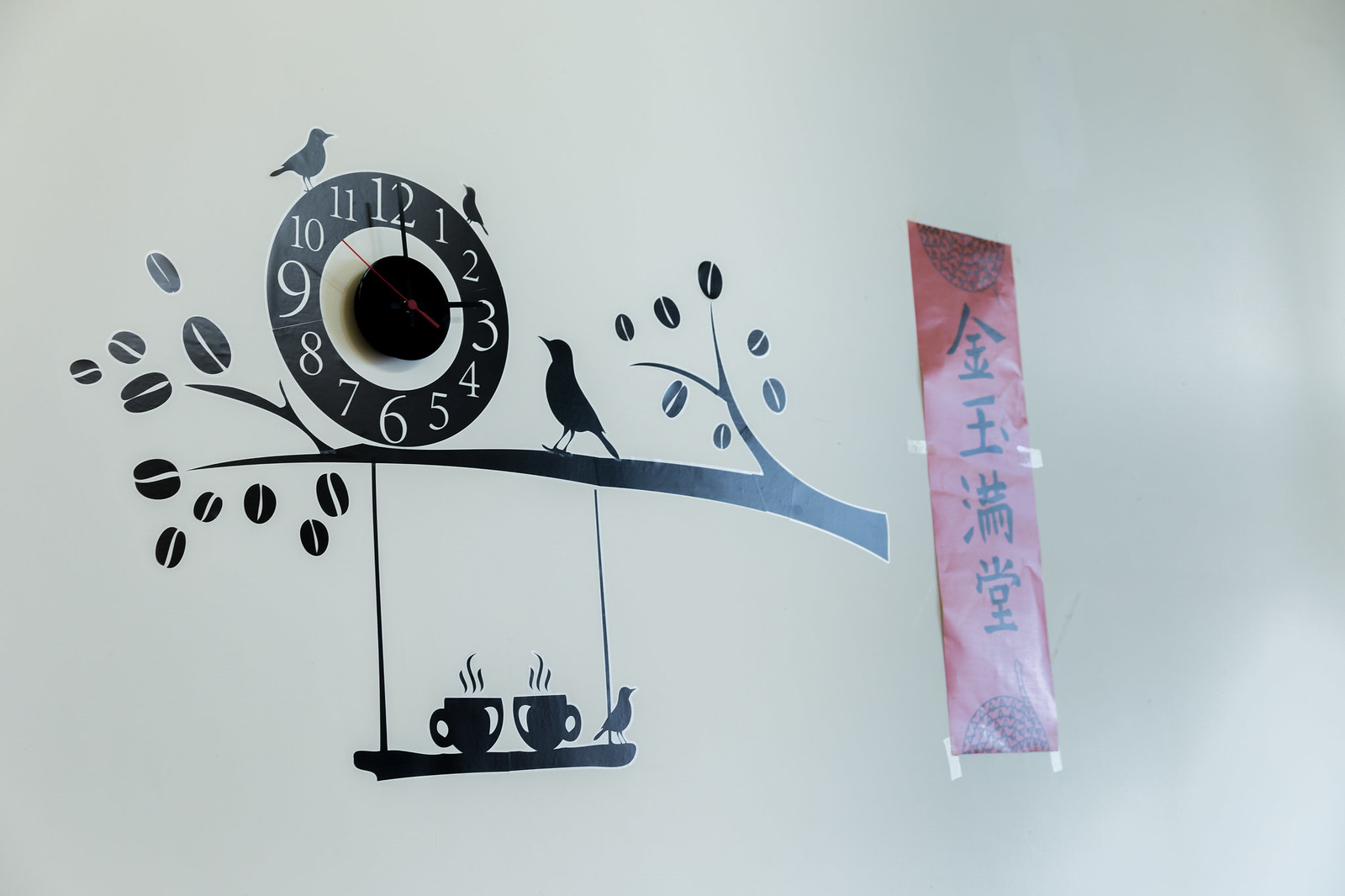The image showcases a unique wall-mounted art installation that integrates a clock into a painted scene on a pristine white wall. The clock itself features a design that resembles a black and white target. The outermost ring is black with white numerals from 1 to 12, inside which is a white circle followed by a smaller black circle at the center. This central black circle houses the hour, minute, and second hands, with the hour and minute hands in black and the second hand in a striking red.

Extending from beneath the clock is a painted branch adorned with black, bean-like leaves. This branch supports two black coffee cups hanging from a swing, adding a whimsical touch to the composition. Additionally, there are a couple of black birds perched on the branch and the swing, enhancing the natural, serene aesthetic of the scene. A red vertical banner with black Asian characters descending upon it adds a cultural and artistic flair to the overall design.